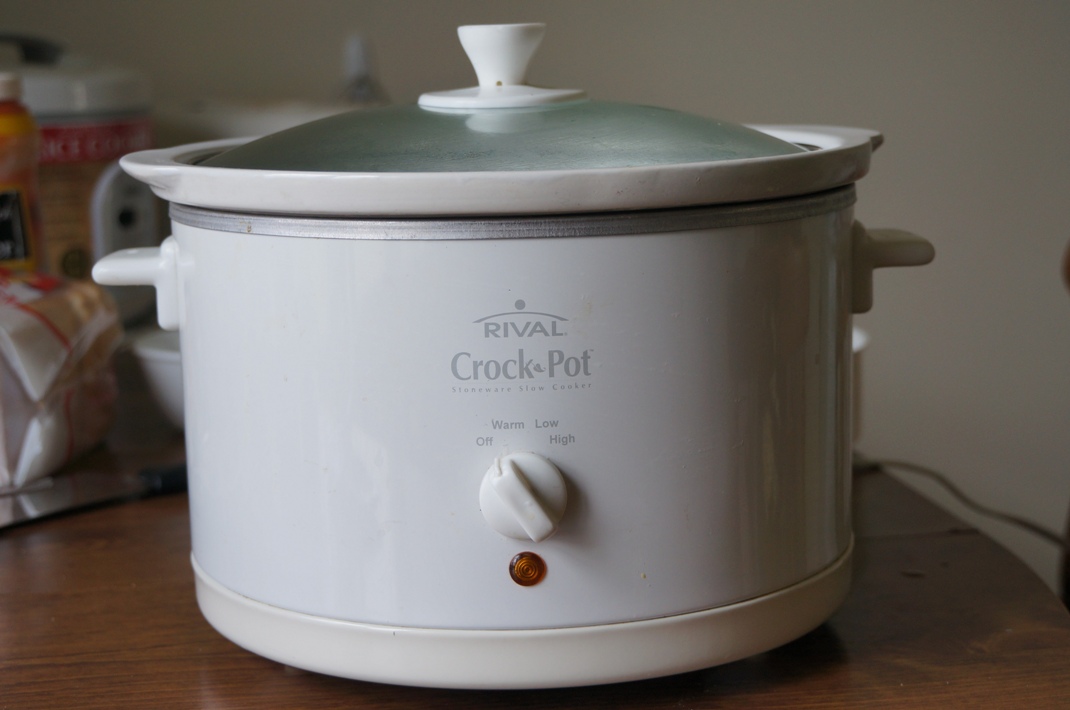The photograph, taken in landscape orientation, captures a close-up of an old Rival Crockpot, which appears to be a model from about 10 to 20 years ago. The crockpot is white, with the brand name "Rival Crockpot" prominently displayed in the center. It features a single knob underneath the branding, marked with settings for 'off,' 'warm,' 'low,' and 'high,' and directly below the knob is a small red indicator light, which is currently off, indicating the appliance is not in use. The crockpot has a circular shape with a glass lid topped with a white handle, looking slightly steamy or cloudy. It also has two side handles for easy lifting. The appliance rests on a table with a rich walnut wood color. The background is slightly out of focus and shows a variety of pantry staples, including a loaf of bread still in its plastic wrapping and a bowl peeking from behind the crockpot. The wall behind the table is a dark cream color, and a power cord extends from the right side of the crockpot, likely plugged into an unseen outlet. The overall muted colors of the photograph give it a vintage feel, reminiscent of the 1980s.